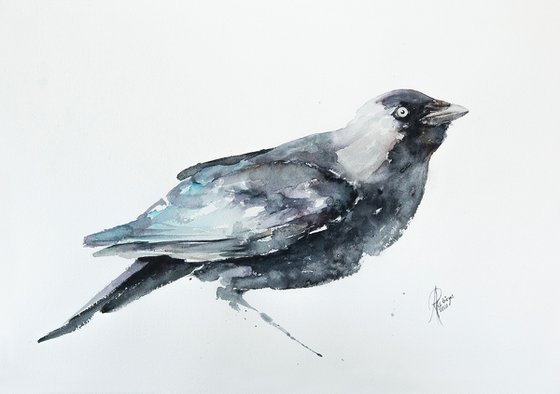This image is an intricate watercolor painting of a bird, likely a blue jay, facing towards the right. The bird, occupying the center of the image, is illustrated in various shades of blue, gray, black, and white. The head, a mix of dark gray and black, features a striking white eye with a black pupil, and a light greenish-gray beak. The neck and upper back display a patchwork of white, transitioning into a blend of blue, gray, and lighter colors on the wings. The tail, darker at the bottom and lighter at the top, extends towards the bottom left corner of the image. The entire composition sits against a light gray or off-white background, with the suggestion of a light source from the upper left corner adding depth to the bird's form. The illustration is signed by the artist in cursive at the bottom right, adding a personal touch to this captivating portrayal.